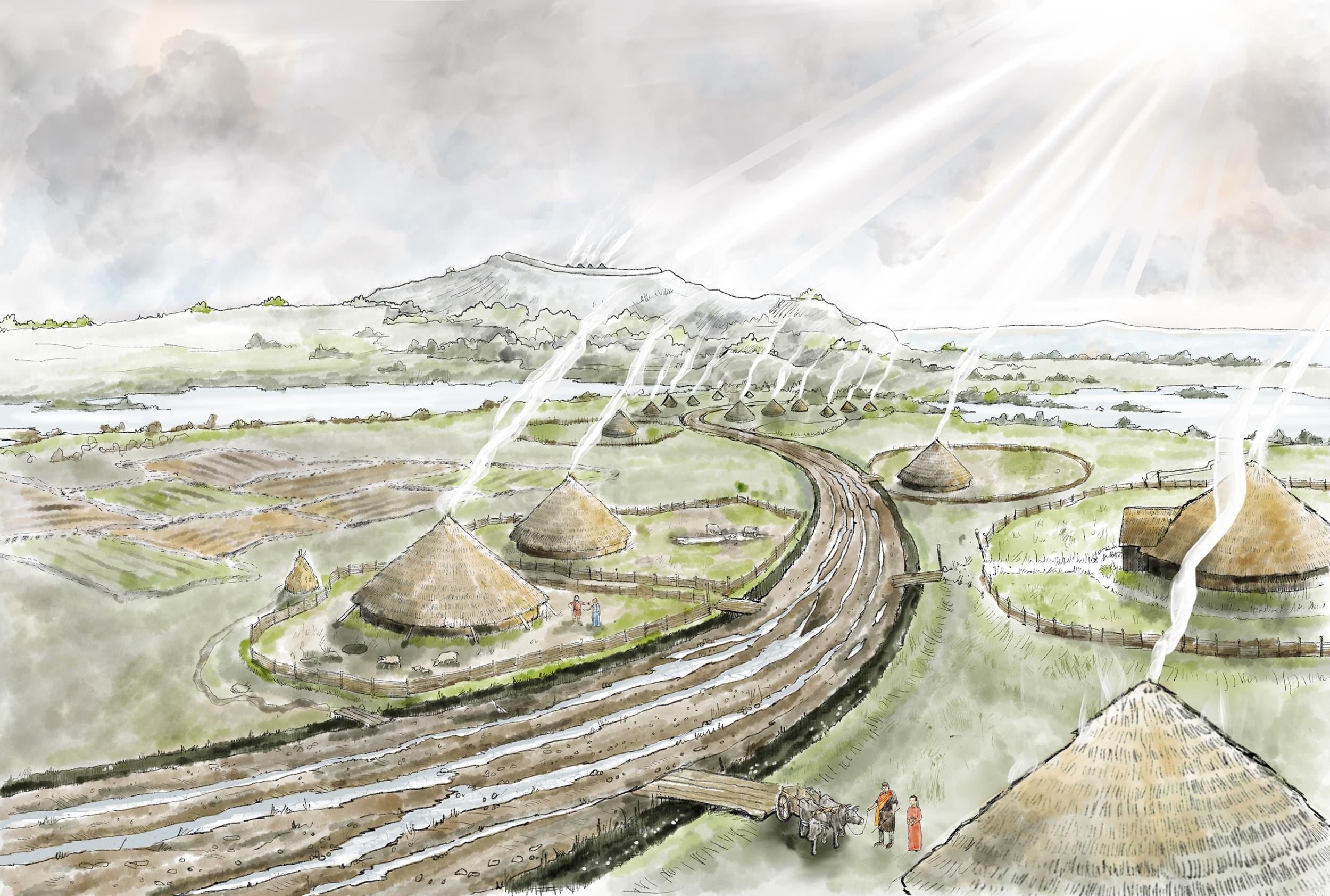This detailed artwork or sketch depicts a vibrant rural scene, possibly inspired by Central Asian or Mongolian settings. The focal point is a collection of traditional yurts with low walls and high conical, thatched roofs, each emitting white smoke from their tops. These yurts are surrounded by large circular corrals or fenced-in areas. 

In the central part of the image, a dirt roadway meanders through the scene, flanked by green grass, and serves as a bridge over small water bodies. A man and a woman, with the latter dressed in an orange dress, stand next to a team of oxen pulling a wooden cart near this road. Additional wooden plank bridges connect each yurt to the dirt road, indicating a network of pathways.

The background features a gray, cloudy sky with beams of sunlight piercing through, illuminating a distant gray mountain. This landscape includes fields, trees, and a serene ambiance that blends both natural and human elements harmoniously. The entire artwork, which appears to be a combination of line drawing and watercolor, captures a snapshot of pastoral life with intricate details and dynamic interactions between people, animals, and nature.